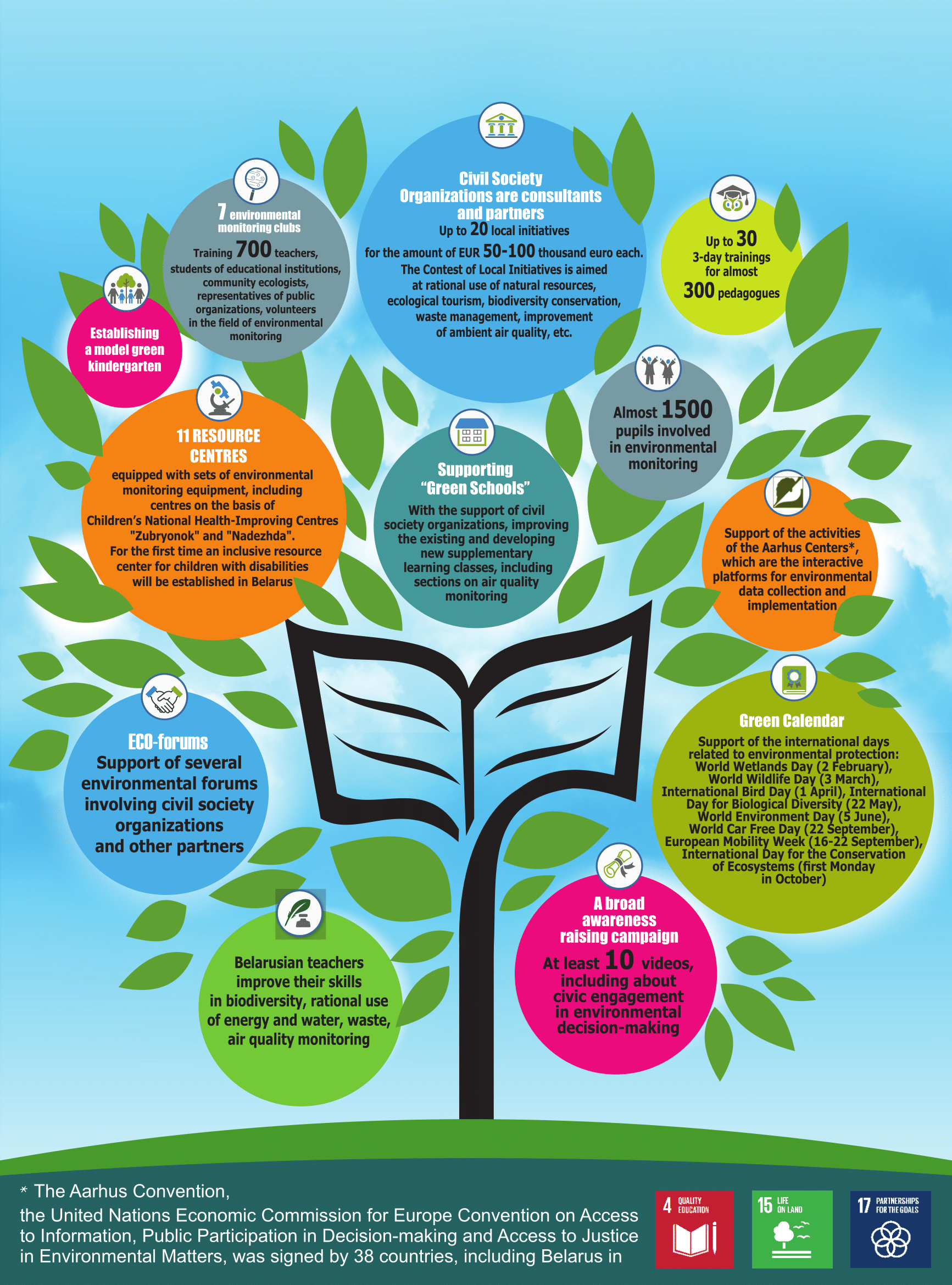This is a detailed poster centered around environmental education and involvement, designed in the shape of a tree growing from an open book, symbolizing knowledge and growth. The background at the top is blue, transitioning to a green oval or hill shape at the bottom, where the tree trunk starts. This black tree trunk rises and branches into open pages scattered with green leaves, each adorned with large and small colored circles resembling fruit. These circles contain information about various initiatives and accomplishments related to the Art Huss Convention, part of the United Nations Economic Commission for Europe Convention on Access to Information, Public Participation in Decision Making, and Access to Justice in Environmental Matters, signed by 38 countries including Belarus.

Each circle represents a specific piece of information or statistic about the convention’s impact and goals. Examples include numbers of local initiatives, training programs for educators, and student involvement in environmental monitoring:

- A blue circle indicating almost 15,000 pupils involved in environmental monitoring.
- An orange circle mentioning up to 30 three-day training sessions for nearly 300 pedagogues.
- Another circle highlighting civil society organizations as consultants and partners.

At the bottom of the poster, against the dark blue footer with white text, the convention's formal title is printed clearly. Below this text and to the right, there are three colored squares—red, green, and blue—with smaller, blurred white print and images that are difficult to discern. The overall visual is engaging and colorful, meant to attract attention and convey comprehensive details about the convention’s initiatives and achievements in promoting environmental awareness and participation.